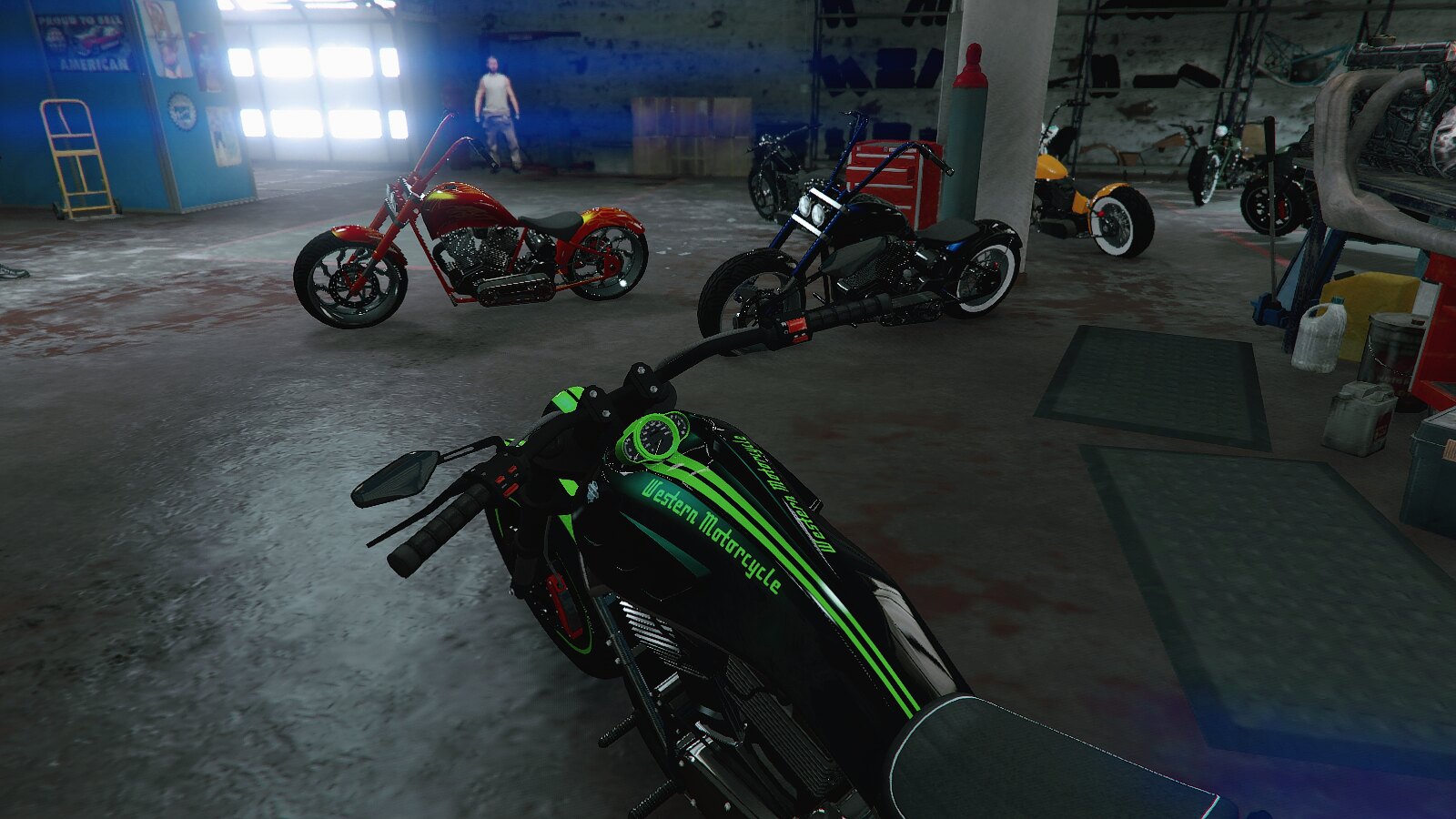The image depicts a dimly lit, large garage or repair shop with a concrete floor. Bright light streams through windows in the garage door, partially illuminating the scene. At the forefront, a black motorcycle with distinctive yellow pinstripes and the words "Western Motorcycle" in green is prominently displayed. Surrounding it are several more motorcycles: a red one with a black seat, a black one with double headlights, an orange and black one with thick white-walled rear tires, and additional dark motorcycles receding into the background.

The garage features various equipment and furnishings, including a red mechanic's chest, red toolboxes, gray mats, throw carpets, and some shelves along the walls. A notable piece of equipment is a yellow dolly cart, used for transporting items. There's also an indistinct figure of a man, likely Caucasian, standing far back in the scene, wearing a white t-shirt and blue pants, partially obscured due to the low lighting. Additional details include a large floor jack and some paintings on the back walls, contributing to the garage's typical cluttered yet organized atmosphere, punctuated with a sense of active vehicle maintenance and repair.